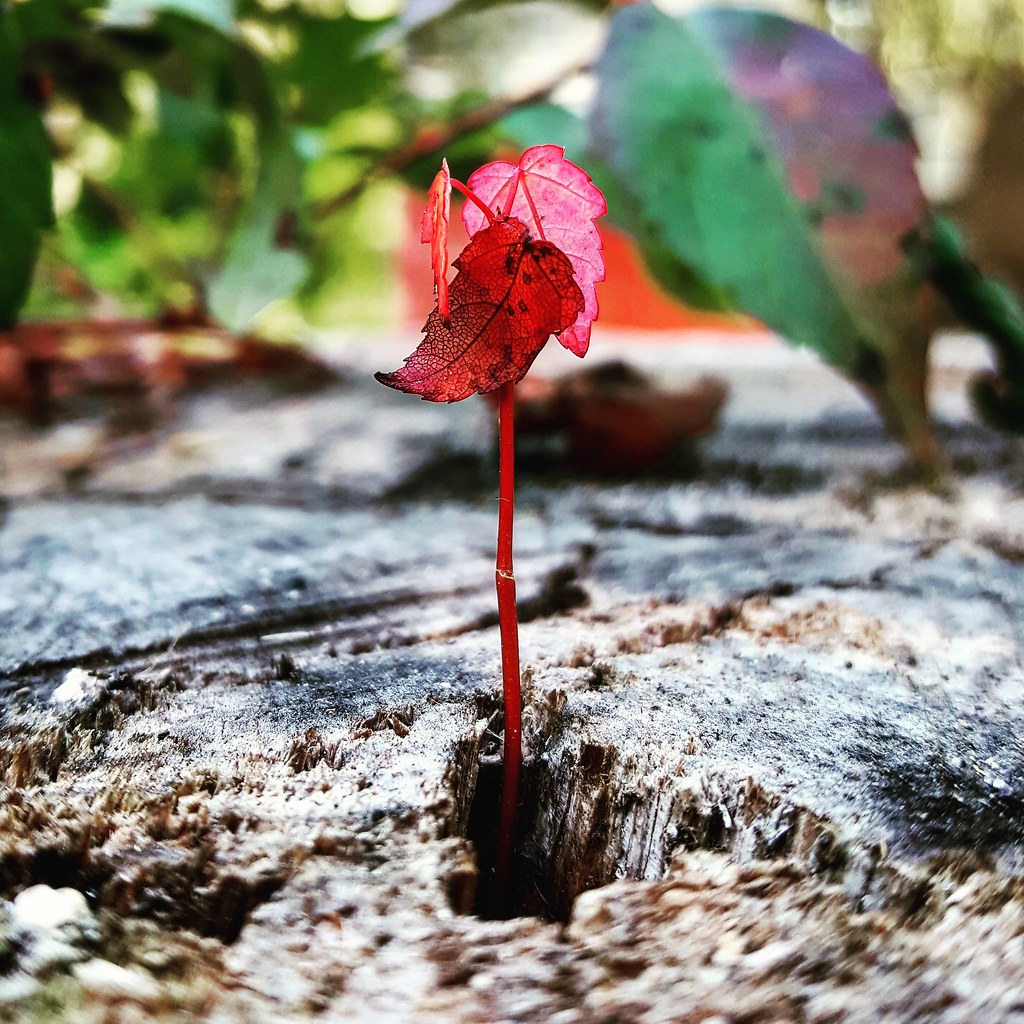An up-close photograph captures a vibrant red plant emerging resiliently from what appears to be the splintered and segmented trunk of a tree. The ground, a mix of wood and bark, reveals a rough, almost sunlit surface with holes, through one of which the plant seems to defy its environment by shooting up. The plant features a slender, bright red stem with three red leaves tinged with pink hues and dotted with black spots. The backdrop displays a blurred array of green foliage with hints of red, bringing additional contrast to the already striking red plant. The overall scene, devoid of people or text, suggests an outdoor setting, possibly in autumn, as signified by the vibrant leaf colors.